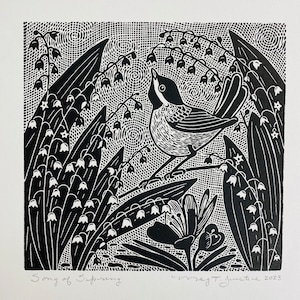The image depicts a meticulously detailed black and white artwork, possibly created through a technique such as weaving or needlepoint. Central to the piece is a bird perched on a branch, its beak angled upwards. The bird features a distinctive coloration: a white and grey belly, black and white striped wings, a black head with a white stripe extending from the back of its head to the tip of its sharp black beak, and a stripe beneath its eye. Surrounding the bird are large, black leaves accented with white veins and smaller flowers in varying shades of white and black, some of which resemble delicate bluebells. These flowers arch elegantly across the canvas with one prominent large flower located beneath the bird. The background is filled with intricate swirly patterns, composed of lines and small dots, adding to the overall complexity of the drawing. At the bottom of the image, there is a cursive inscription that partially reads "Song of Sympathy" and another partially legible phrase, suggesting the artwork may be signed with "Métis something 2024." These details collectively create a rich and captivating visual narrative.